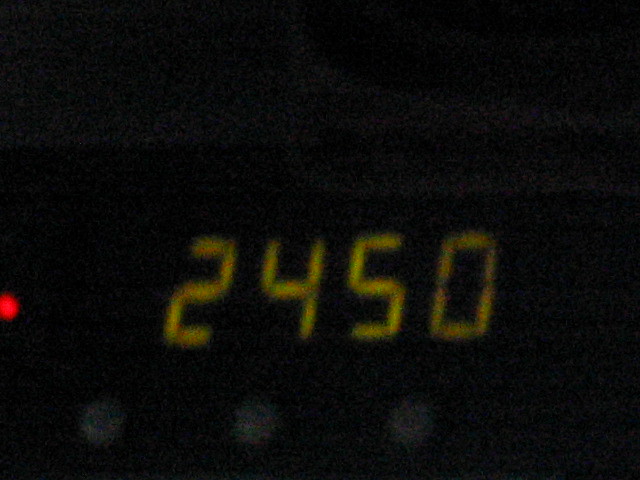This image is a color photograph featuring a predominantly pitch-black background, giving it an overall dark appearance. At the center of the bottom third of the image, there is a digital display showing the glowing yellow numbers "2450," possibly indicating a time or measurement in the manner of a digital clock or calculator. On the left side of the image, about three-quarters of the way down, a round red dot is illuminated. Beneath the digital display, three small, light gray, and slightly blurred spots are visible, resembling possible buttons or controls. The photograph is slightly grainy and out of focus, making it difficult to determine the exact nature of the device.